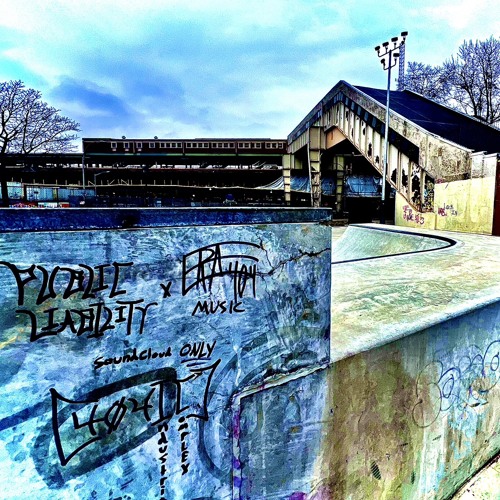This daytime photograph captures an abandoned train station, prominently featuring an old structure with stairs likely leading to a subway platform. The main focus is an extensive graffiti-covered wall, with some legible text like "music" or "SoundCloud" amidst various unclear tags. The scene is set during winter, evidenced by the leafless trees in the background. Surrounding the station are stadium lights and dilapidated buildings with broken windows. To the left, there is a graffitied wall, while the right side shows a sloping path under a bridge with steps leading up to it. The overall image has a slightly gloomy appearance, enhanced by a blue-tinted filter and sparse clouds in the sky, giving it a cool, almost surreal vibe.